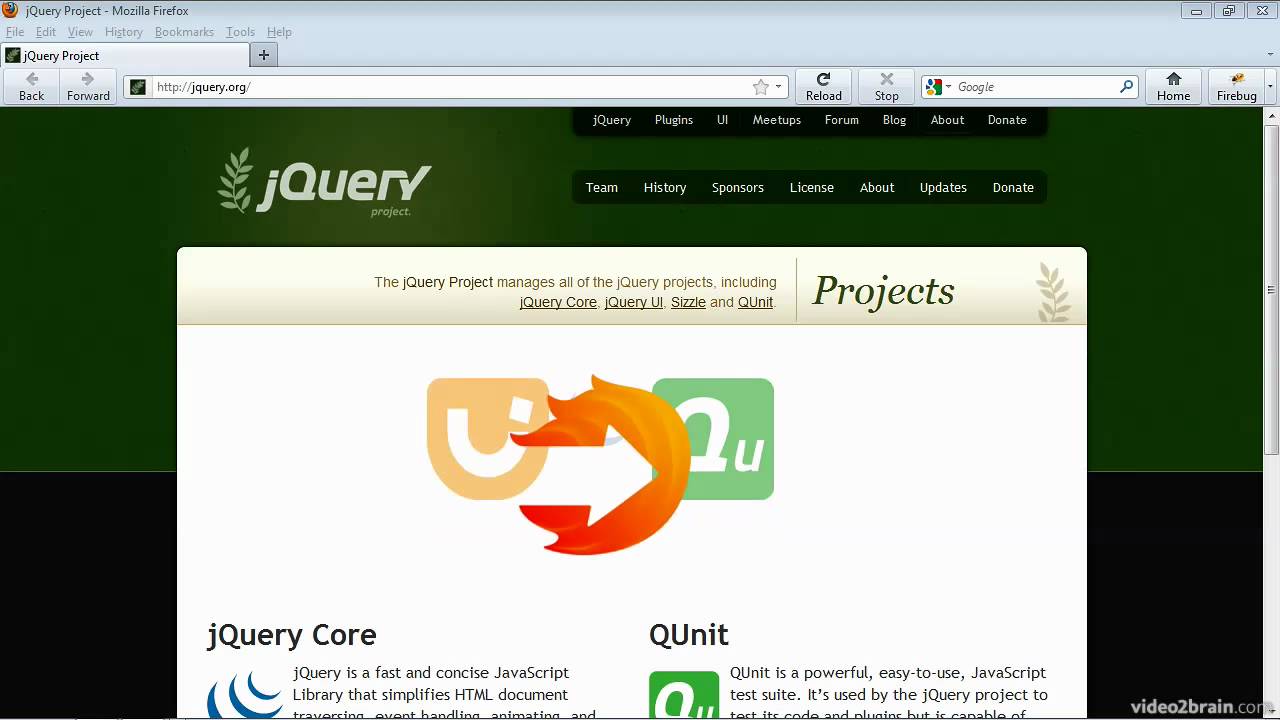This image is a screenshot of a webpage from jquery.org, clearly showing the browser's top section, including the web address. The website features a two-toned background: the upper half is dark green, and the lower half is black. At the top of the page, the jQuery logo is prominently displayed—a small "j" followed by a capital "Q" and then "uery" written in gray. To the left of the logo, there's a simple illustration of a branch with leaves. To the right of the logo is the main navigation menu, with the options "Team," "History," "Sponsors," "License," "About," "Updates," and "Donate" all presented in white font against the black background.

Below the header, there is an off-white rectangular inset with a banner reading, "The jQuery project manages all the jQuery products including jQuery Core, jQuery UI, Sizzle, and QUnit." 

In the center of the screen, there's a large diagram prominently featuring a white letter "U" inside a light pink square. Adjacent to this is an orange element with an arrow pointing to the right, leading to a green square with rounded corners marked with the text "QU."